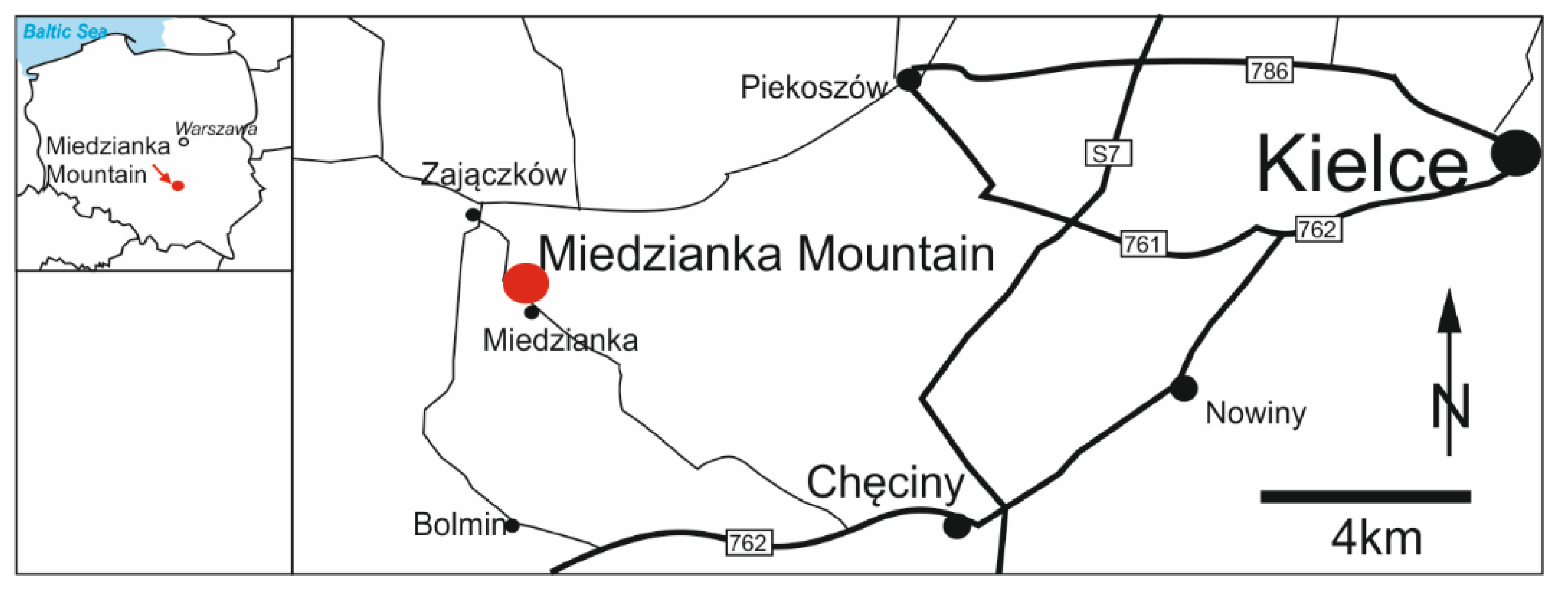This black-and-white map prominently features a zoomed-in area likely in Poland, indicated by the Polish language on the map and the relation to Warsaw. The central focus of the map is Miedzianka Mountain, marked with a red dot and highlighted by a red arrow on a smaller inset map in the top left corner, which also shows the Baltic Sea in blue. The main portion of the map details various roads, including 762, 761, S7, and 786, linking towns with names difficult to pronounce. Notably, there's a compass arrow pointing north in the bottom right, alongside a black horizontal scale line labeled "4KM."